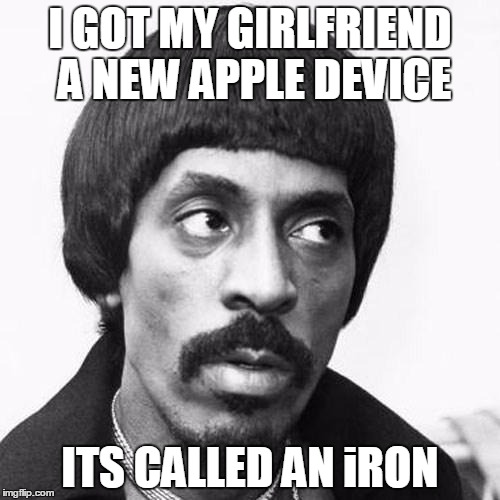This is a black-and-white meme featuring an African American man with a mustache, a slight beard or goatee, and straight, relaxed hair styled into a bowl cut. His hair is brushed down and cut right at his forehead, leaving little space between his eyebrows and his hairline. He is wearing a dark shirt or possibly a coat, with hints of gold chains around his neck. The man is looking up and to the left with a neutral expression, his mouth slightly open. The background is light gray and somewhat blurry, creating an indistinct setting. Overlaying the image, bold white text reads at the top, "I got my girlfriend a new Apple device," and at the bottom, it humorously adds, "it's called an iRON." In the bottom left corner, small text credits the source as IMGFLIP.COM.